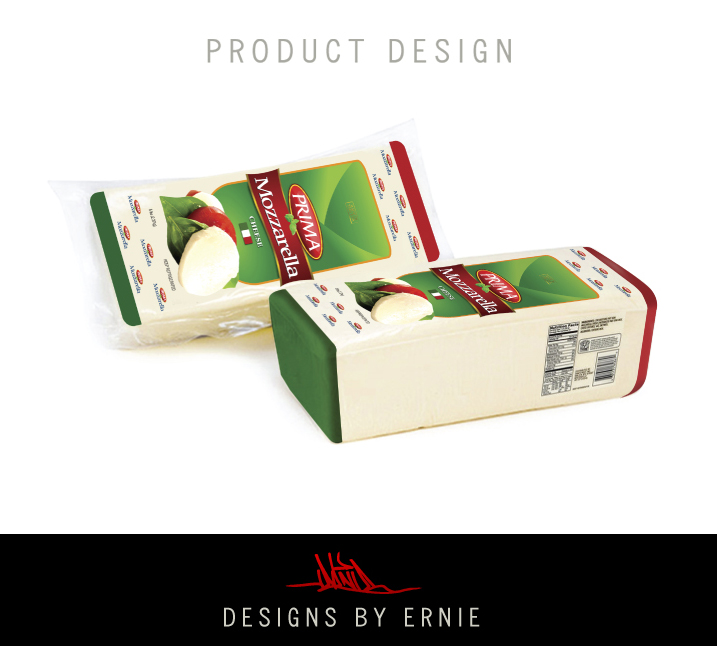The image showcases a detailed product advertisement for Prima Mozzarella Cheese. Central to the image are two representations of the product: one lying flat and another tilted to display more information. Both the box and the actual mozzarella product feature a distinguishing label with a green background and white text reading "Prima Mozzarella Cheese." The packaging embodies Italian colors, with the top part in red, the bottom in green, and the majority of the surface in cream. On the top of the entire image, the text "Product Design" is displayed in gray against a white backdrop. The packages are adorned with the Prima label prominently on the front. Additionally, the visual includes slabs of mozzarella cheese placed next to lettuce and tomatoes, enhancing the appeal of the product. At the bottom of the image, a black horizontal strip contains a logo and the text "Designs by Ernie" in white font. Red text, possibly a signature or logo, accompanies this design. The product presentation aims to effectively communicate the brand and nutritional aspects, though the detailed information remains indistinct.